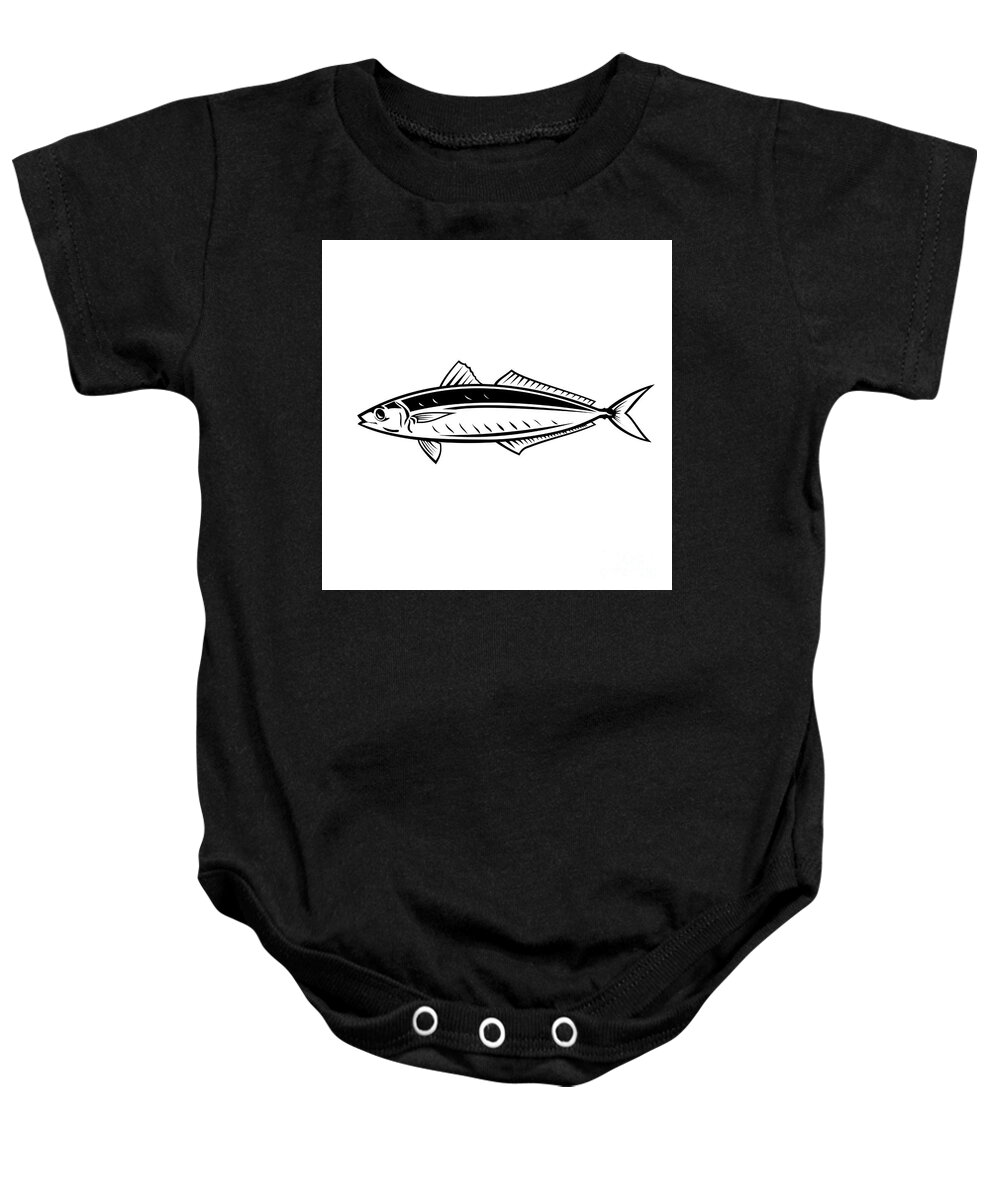This image depicts a black baby onesie with short sleeves and a unique central design. The focal point of the garment is a white square situated in the middle of the chest, featuring a black outline drawing of a fish facing left. The fish illustration includes distinct details such as a black stripe along its back, a set of four gills marked by small black stripes, and a pointy tail. Additionally, the fish has various fins, with a long fin at the top, a shorter one towards the front, and another long fin near the tail end. The onesie is equipped with three silver circular snaps at the bottom in the crotch area, designed for easy diaper changes. The background of the photograph is entirely clear, highlighting only the onesie which is not being worn. No other objects, text, animals, or people are visible in this image.